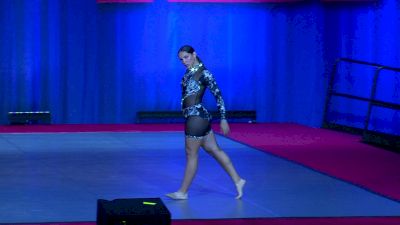In this grainy, slightly blurry photograph, a woman is captured walking on a blue gymnastics mat, bordered by red. She’s wearing a black one-piece gymnastics outfit that ends in shorts and has long sleeves, decorated with blue lines and silver sparkles. Her dark hair is pulled back into a ponytail. She is barefoot, and there seems to be a hint of white chalk on her feet, emphasizing her role as a gymnast. Her left hand hangs by her side while her right hand is out of frame. The backdrop includes blue curtains and a dark blue wall with a railing. There are visible speakers in the front and upper left corner of the image. The woman appears to be walking towards the center of the mat with a determined look, suggesting she is focused and ready for her routine. The overall image, likely taken from an old phone or camera, has a nostalgic, grainy quality.